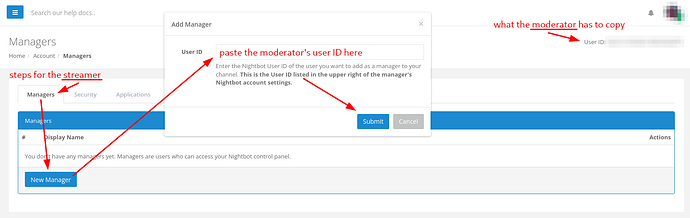This image displays a screenshot of a webpage dedicated to managing user permissions, specifically for adding managers via a help documentation interface. The main heading, "Search Our Help Docs," is prominently featured at the top. Below it, breadcrumb navigation reads: "Home / Account / Managers," indicating the specific section being viewed.

The focus of the page is the "Managers" section, where an interactive element for adding a new manager is present. A user has clicked on the "Managers" section, causing a popup form titled "Add Manager" to appear. This form includes a field labeled "User ID" with the instruction, "Paste the moderator's user ID here," highlighted in red. 

There is an annotated red arrow pointing from the text "New Manager" to the "User ID" field, emphasizing where the user ID should be input. Another red arrow guides the viewer from the word "Listed" to the "Submit" button, which is part of the process of submitting the new manager's information. An explanatory note reads, "Enter the Nightbot User ID of the user you want to add as a manager to your channel. This is the user ID listed in the upper right of the Manager's Nightbot account settings."

To the right of the form, there is a "Cancel" button for users who choose not to proceed with the submission. Additional red text explains what the moderator needs to copy, with an underlined "Moderator" and an arrow pointing to the "User ID" field, underscoring the importance of this step.

For privacy, the user ID field has been blurred out, as indicated by the blurred ID and an icon above it. The webpage predominantly features blue tones, with white text and strategic use of red for emphasis and guidance.